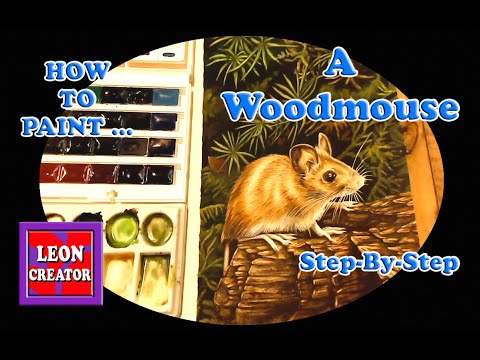This detailed title card for a tutorial video features the text "How to Paint a Wood Mouse Step-by-Step" prominently in blue with a white outline. Set against a black background, the central focus is a detailed oval illustration of a brown wood mouse with a white belly and whiskers, perched on a fallen log. Surrounding the log are green pine needles, trees, and leaves, enhancing the natural scene. A purple square with white text in the lower-left corner reads "Leon Creator," adding a personal touch from the creator. Additional red splotches provide contrast to the composition. The overall design is visually engaging and hints at the step-by-step painting instructions to be followed in the tutorial.